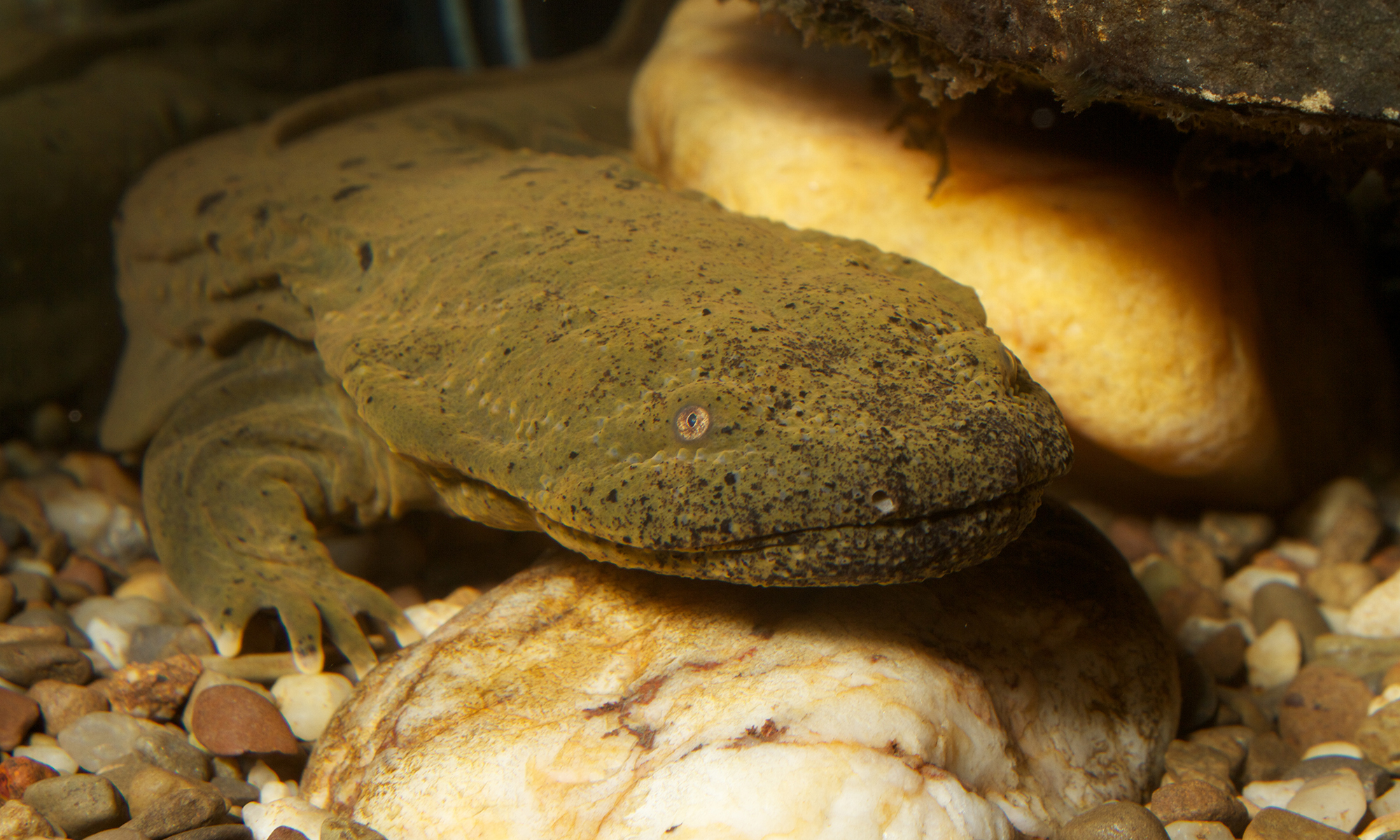The image captures a detailed close-up of a gray-brown lizard, possibly underwater, blending with its environment. The scene is filled with various rocks and pebbles, creating a natural setting. The lizard, partially submerged, has a speckled gray-brown body with small black dots that provide excellent camouflage against the sediment-like backdrop. Its tiny eyes, which almost match its body color, have protective lenses and beady black pupils. Its mouth is wide and circular, though closed in this image. The reptile is resting on a prominent white rock with several cracks and dark brown spots, surrounded by smaller, smoother pebbles in shades of black, brown, tan, gray, and white. Vegetation is seen growing on a dark gray rock in the top right corner. The lizard has four fingers on its visible claw and a ridge running along its back. The scene suggests an underwater habitat rich with details, creating a vivid nature-themed photograph.